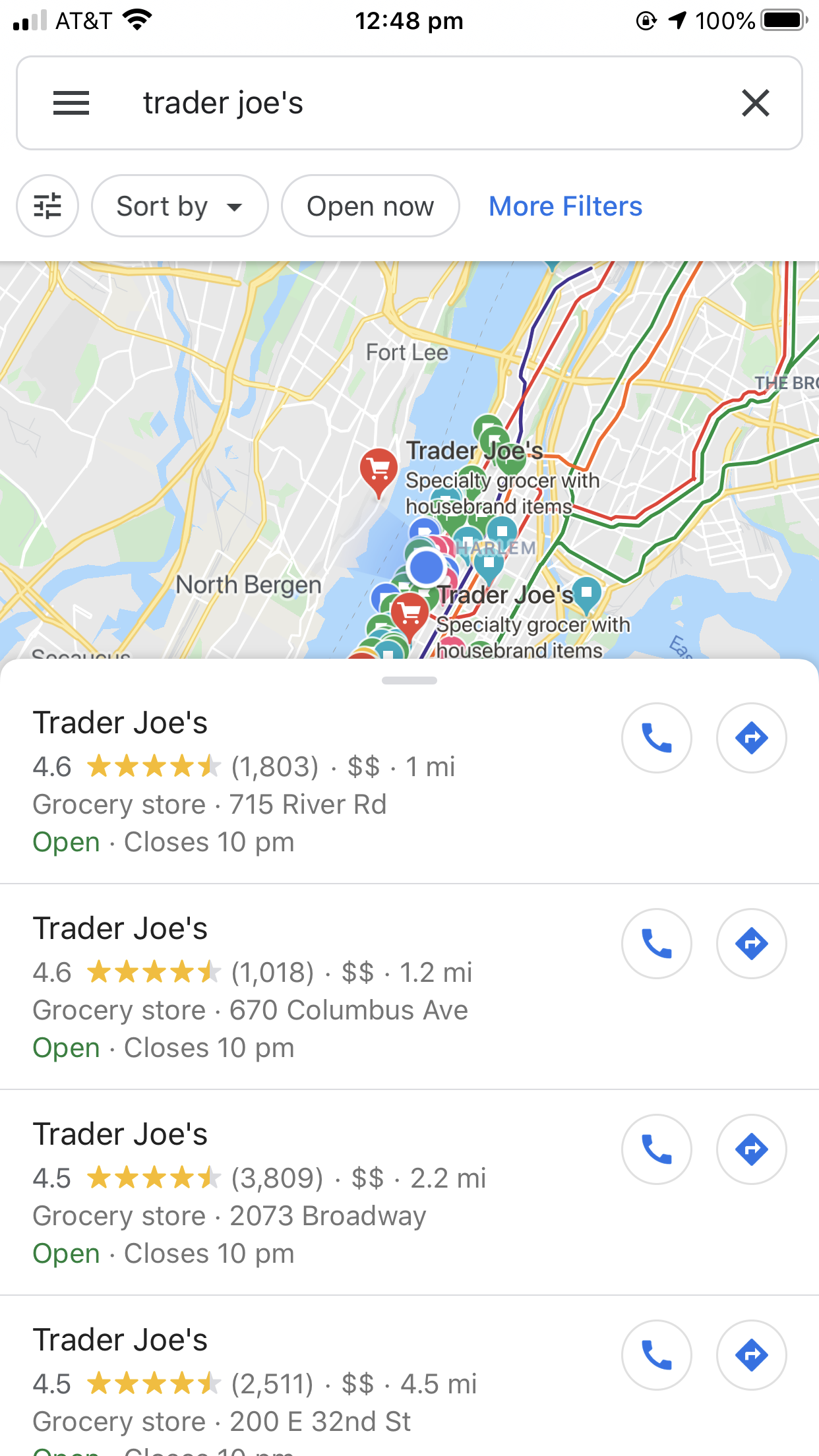The screenshot depicts a Google Maps search interface on a smartphone. At the top-right corner, the status bar shows a battery level at 100%, the current time of 12:48 p.m., and the carrier information with AT&T and a Wi-Fi signal icon on the left. Below the status bar, there is a search bar with "Trader Joe's" entered, alongside an 'X' button for clearing the search term.

Directly underneath the search bar, there are filtering options including a circular filter icon, a bubble labeled "Sort by," a bubble indicating "Open now," and a blue link labeled "More filters." 

The main display area then features a map showcasing cities such as North Bergen, Fort Lee in New Jersey, and several locations in Manhattan. Under the map, a list of four Trader Joe's search results is displayed. The locations are:

1. **715 River Road,** which is 1 mile away.
2. **670 Columbus Avenue,** which is 1.2 miles away.
3. **2733 Broadway,** which is 2.2 miles away.
4. **200 East 32nd Street,** which is 4.5 miles away.

Each search result entry includes two icons: a blue phone symbol and a diamond-shaped icon with a right-pointing arrow, presumably for calling the store and getting directions, respectively.